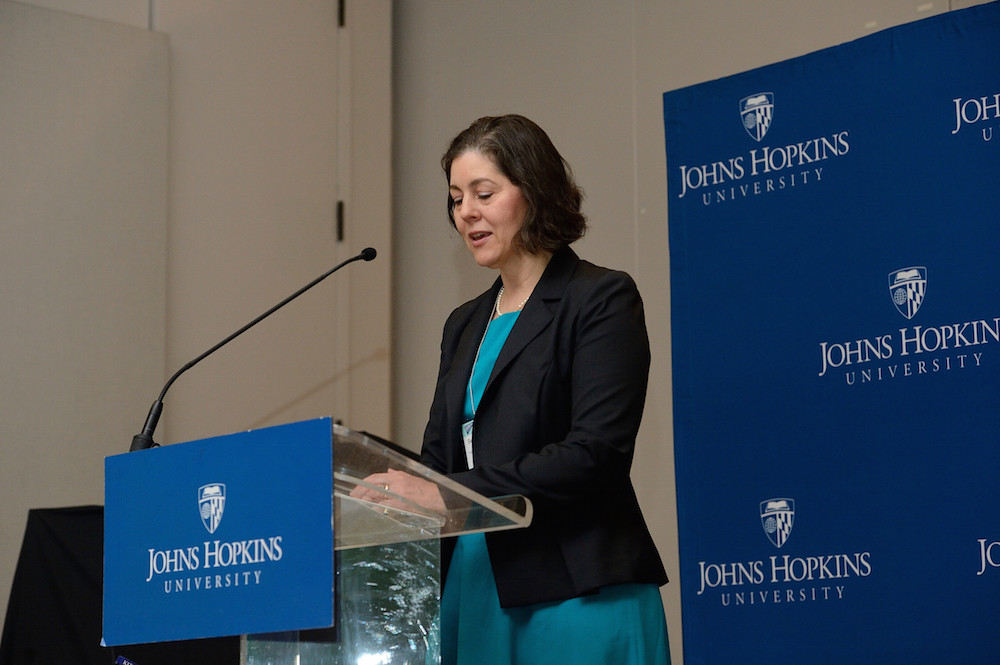In this image, a mid-40s Caucasian woman with chin-length dark wavy brown hair, parted at the side, is seen standing behind a clear acrylic podium. She is wearing a black blazer over a light blue or turquoise dress and appears to be delivering a speech, as her mouth is open and she is looking down at her notes. A black stick microphone with a round black head is positioned towards her face. On the front of the podium, there is a prominent blue sign with white text and a logo that reads "Johns Hopkins University." The background features a dingy white wall that appears somewhat dark, but directly behind the speaker, there is a large blue banner, also displaying "Johns Hopkins University" in white letters across multiple areas. This setting suggests an indoor lecture or formal event hosted by Johns Hopkins University. The photograph is rectangular, wider than it is tall.